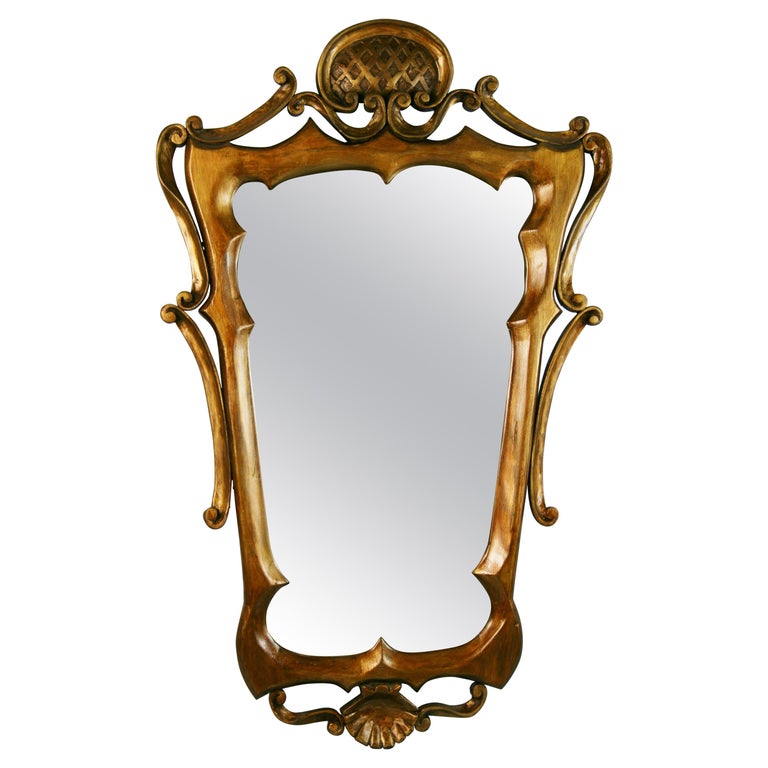The image depicts an ornate, antique mirror with a bronze-colored frame, which exudes a sense of aged elegance. The mirror itself is an elongated vertical rectangle, approximately four feet tall, with a series of intricate designs including spiral, S-shaped swirls along the sides, and flat, mushroom-like shapes at both the top and the bottom. The frame is gold but has a slightly tanned, mid-brown hue that gives it a reflective, almost brass-like appearance. The elaborate frame also features arches and shell motifs, further enhancing its antique look. The glass of the mirror is somewhat cloudy, adding to its vintage charm, and no background details are visible, emphasizing the product-like style of the image.